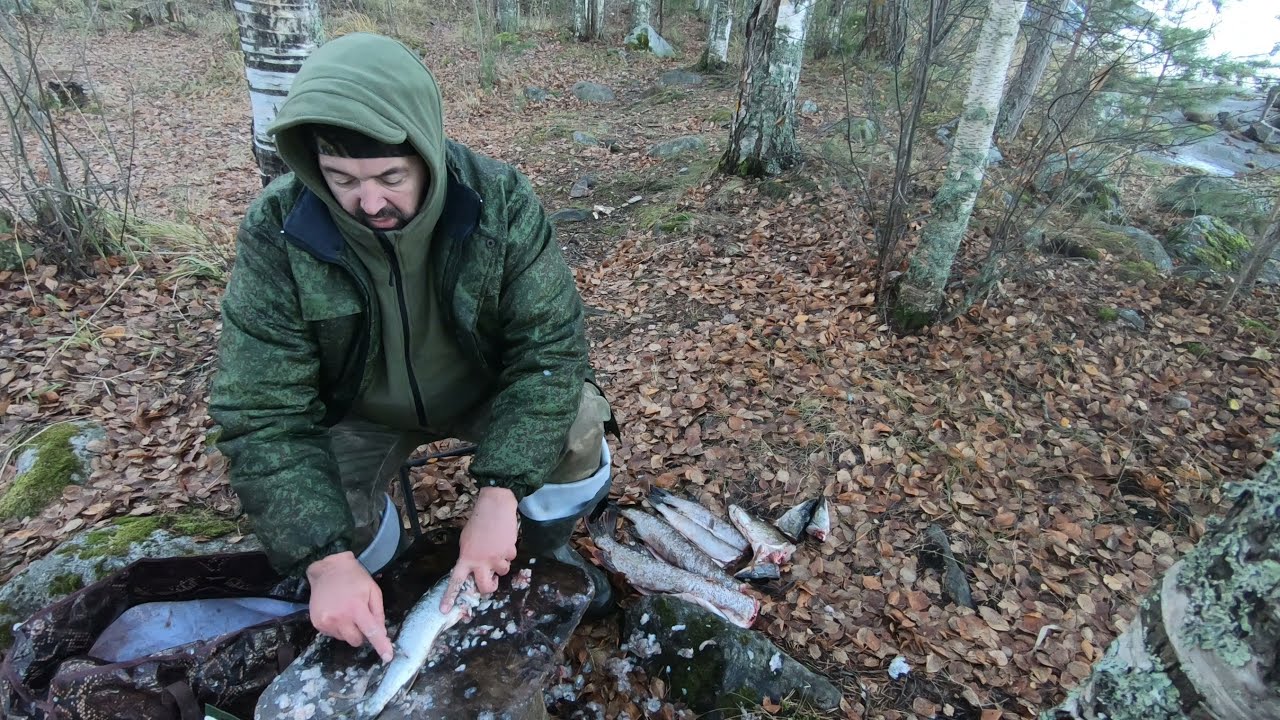In this detailed image, a solitary fisherman is engrossed in cleaning his catch amidst a serene, overcast day in a wooded area. The man, crouched on the left side of the frame, is clad in a green camouflage jacket with an olive green hooded sweatshirt underneath, complemented by greenish-gray pants and rubber boots. His focus is entirely on the task at hand, as he uses a knife to clean a silver-colored fish on either a tree trunk or a rock that serves as his makeshift work surface. Surrounding him, the ground is blanketed with dead leaves, suggesting it might be fall or early winter, though there is no snow. Scattered around his feet are several other fish, some already cleaned, evidence of his diligent efforts. The background is a vista of tree trunks, visible only up to a certain height, enhancing the secluded and tranquil atmosphere of the scene.